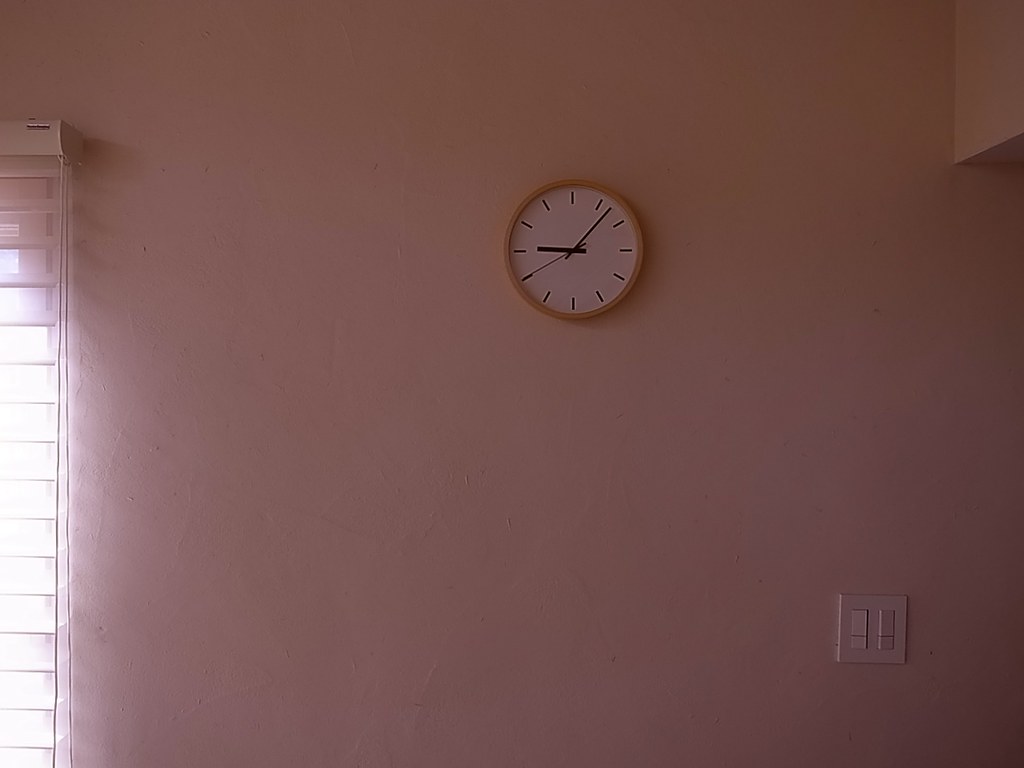The photograph captures an indoor scene featuring a minimalist round clock mounted on a shadowy, beige-colored wall. The clock, which has simple and straight hands, features a face of pristine white encased in a light-colored wooden border, adding a subtle touch of elegance. Nearby on the wall, a beige light switch panel is partially visible. Horizontal blinds on an adjacent window are open, permitting bright sunlight to stream into the room, casting a mix of light and shadow across the space.